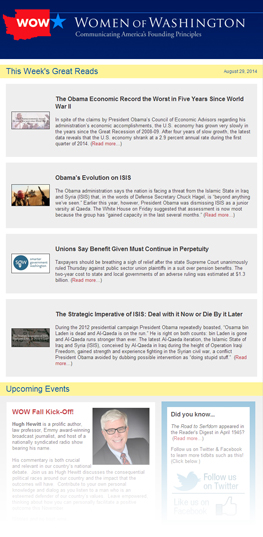This image is of low quality, characterized by its blurriness, fuzziness, and small, hard-to-read text, giving it a somewhat pixelated appearance. In the top left corner of the image, there is an outline of the state of Washington colored in red, with the acronym "WOW" inscribed in white. Adjacent to this, towards the right, is a light blue star set against a dark blue background. The phrase "Woman of Washington" is visibly written, followed by the tagline "Communicating America's Founding Principles." Below this, the text "This Week's Great Reads" appears, accompanied by the date "August 29th, 2014" on the right side.

In the section beneath this header, a title reads, "The Obama Economic Record: The worst in five years since World War II." There is a block of black text under this title, which is unfortunately too small to decipher due to the poor image resolution. Further down, another section is titled, "Obama's Evolution."